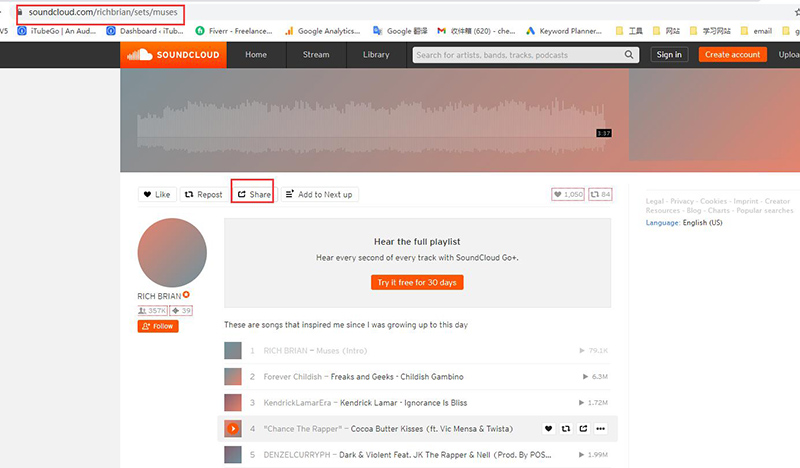This image is a screenshot from the SoundCloud website, captured in a landscape orientation. The screenshot is slightly wider than it is tall. At the top of the image, there's a grey search bar displaying the URL: "soundcloud.com/richbryan/sets/muses".

Beneath the search bar, there's a white border containing a row of the user's favorite icons, including iTubeGo, Dashboard, Fiverr, Google Analytics, Gmail (with some Chinese characters next to it), Keyboard Planner, and additional icons with Chinese lettering.

A horizontal black bar spans the top edge of the webpage. Near its left-center, there's an orange SoundCloud logo featuring a white cloud and the text "SoundCloud" in white. Adjacent to this logo, the navigation options "Home", "Stream", "Library", followed by a search bar, are visible. To the right of these options, there's a black "Sign In" button, an orange "Create Account" button in white font, and an "Upload" option.

Below this, a box features vertical white lines likely representing the song's volume levels. Centrally placed on the page, there's a profile section displaying the name "richbryan", accompanied by a circular icon in shades of pink, purple, and grey.

The main content area showcases a list of five songs, each with options to stream and play them. The layout is clean and organized, focusing on the artist's recent music set.